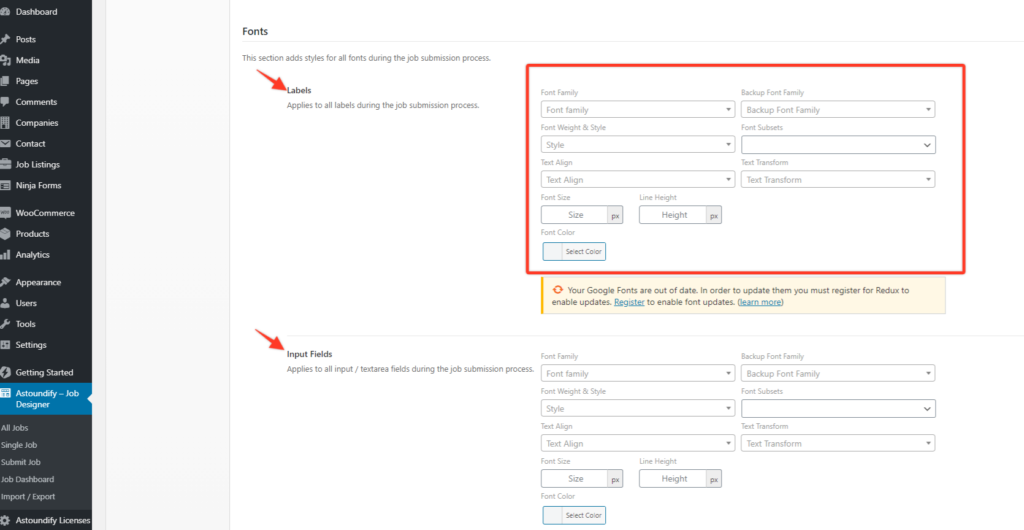In this screenshot, we see a user interface with a predominantly white background, and a black navigation dashboard positioned on the left side. The dashboard is arranged vertically and lists various menu items in white text including: "Posts," "Media," "Pages," "Comments," "Companies," "Contact," "Job Listings," "Ninja Forms," "WooCommerce," "Products," "Analytics," "Appearance," "Users," "Tools," "Settings," and "Getting Started." Below these, in a blue box, is the section titled "Astoundify Job Designer," which is highlighted. Further below, there are additional options: "All Jobs," "Single Job," "Submit Job," "Job Dashboard," and "Import and Export."

To the right of the navigation dashboard, the main area features a white background. At the top left of this section, bold black text reads "Fonts." This section appears to be related to customizing font styles used during the job submission process. A prominent red arrow points to the bolded black word "Labels," indicating that this specific setting applies to all labels displayed during the job submission process. The layout suggests a user-friendly interface designed to facilitate various administrative tasks related to job postings and their associated forms.